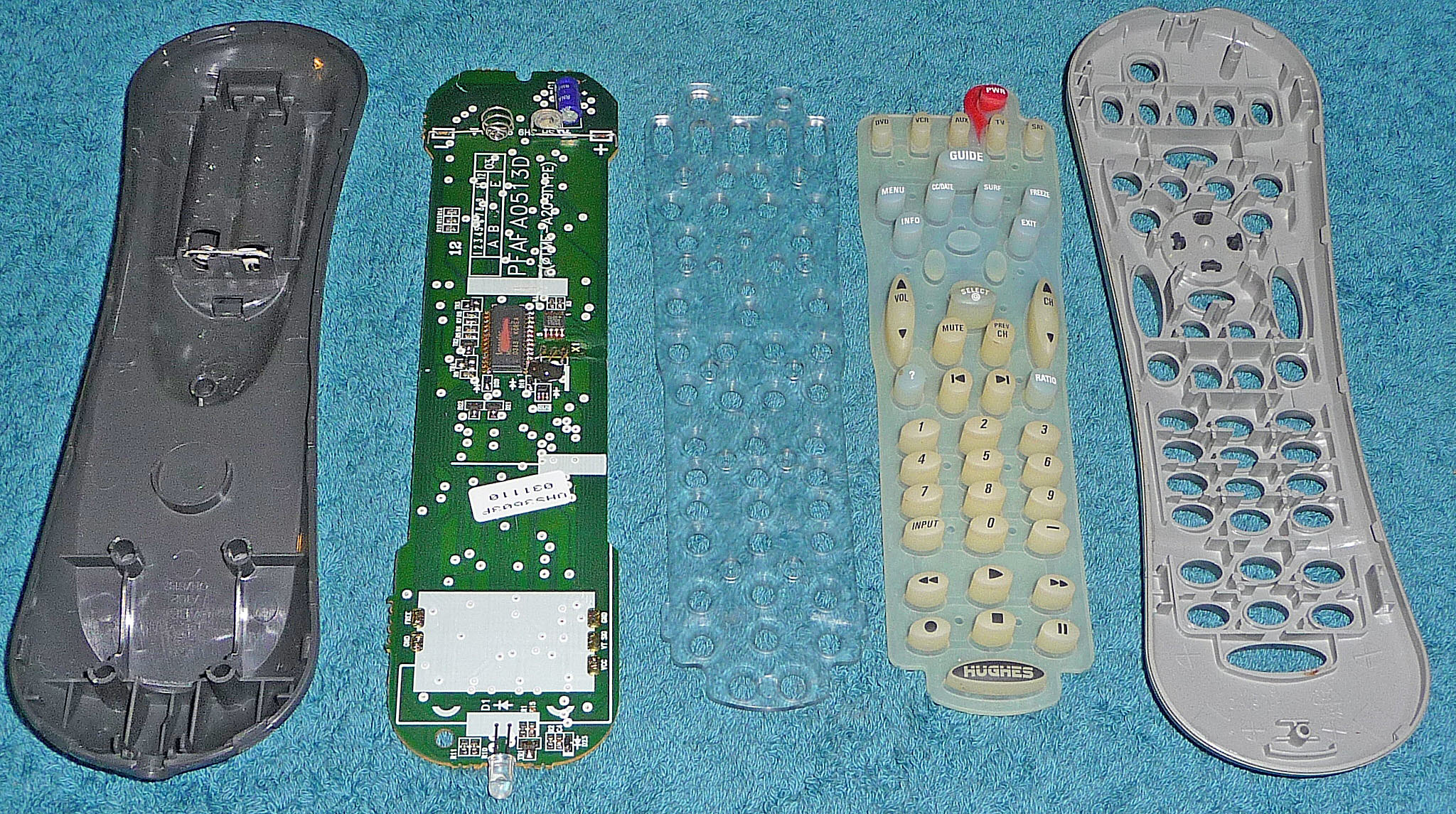The image displays a meticulously dissected television remote control laid out against a soft, light blue fabric background, resembling very short faux fur with darker blue spots. On the far left, there is the dark grey backplate of the remote. Next to it lies the dark green circuit board, featuring an array of wires and tiny silver components that likely react when the remote buttons are pressed. Moving to the middle, there is a clear plastic plate with cutouts designed for the buttons. Adjacent to this, the actual buttons are light tannish-yellow, with a white plastic case; further up, some buttons are light blue, including one labeled "Guide," and there is a distinctive red power button at the top. On the far right, completing the assembly, is the light tan top shell of the remote, aligning the buttons within the housing. This detailed "exploded view" captures each component of the remote, methodically arranged, showcasing the intricate interior and exterior parts.